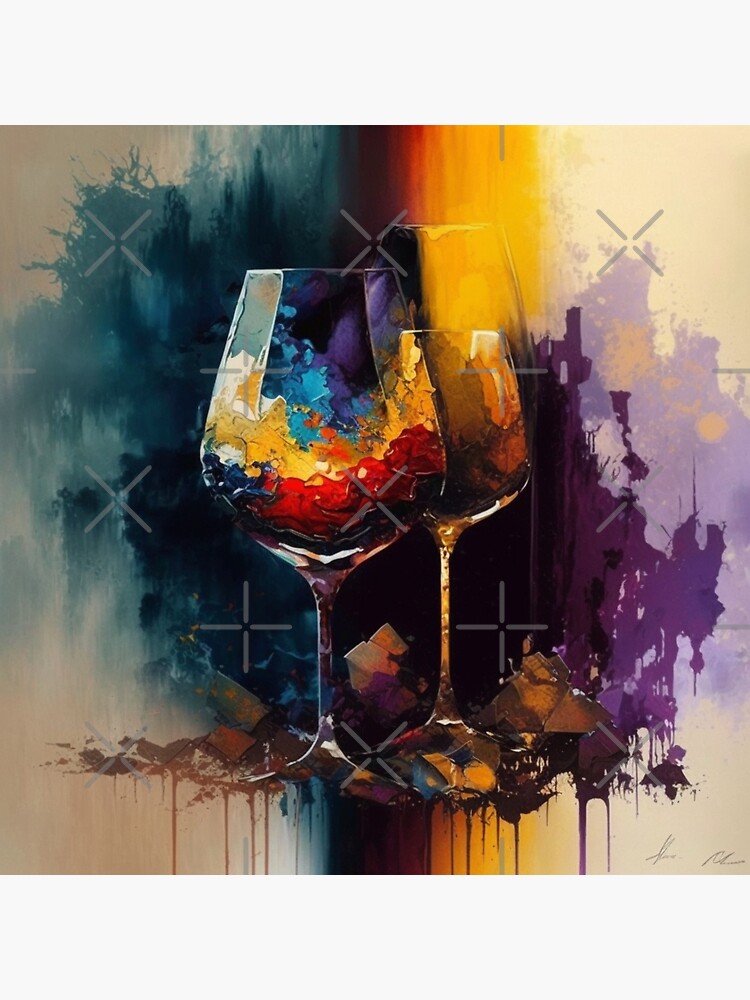This vibrant square painting, likely done in oil or acrylic, depicts two intricately detailed wine glasses positioned centrally against a dynamic abstract background. The wine glasses have elongated stems and varied sizes, with the larger glass on the left and the smaller, goblet-like glass on the right. Within the left glass, layers of vivid colors – red, orange, blue, and purple – appear as if they are liquids, creating a striking, unblended visual effect. The right glass appears to be empty, merely reflecting the surrounding colors. The background comprises broad, dripping splotches of blue, purple, and orange, forming an almost rainbow-like gradient, with colors melding into each other and running down the painting in a melting paint style. This background also includes teal, brown, yellow, and pink tones, contributing to the rich, fluid ambiance of the artwork. Superimposed over the painting is a repetitive gray X and plus watermark pattern, imparting a unique texture to the image. The edges of the painting are bordered by an inch-thick white frame, enhancing its presentation.